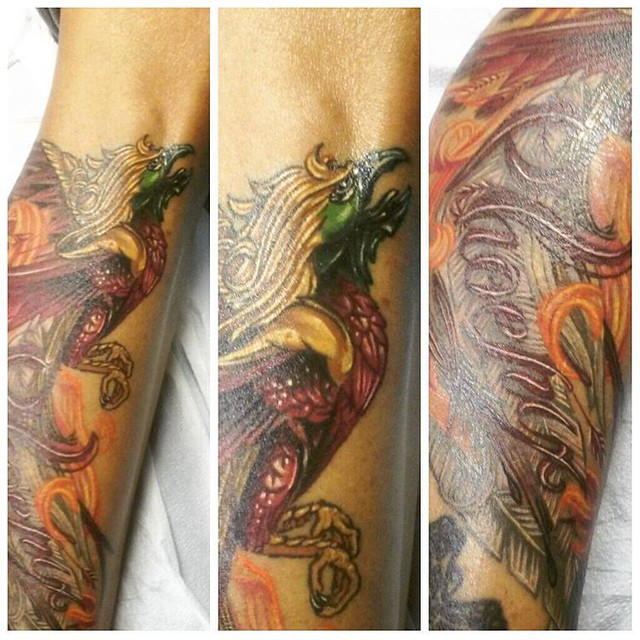The image is a composite of three close-up photographs showcasing a detailed tattoo on a person's forearm. The tattoo depicts a striking phoenix with an open beak and large, raptor-like claws, launching upward in a dynamic pose. Its vibrant colors include a bronze body, a green face, and fiery, hair-like feathers flowing from its head. Pink feathers adorn its chest, and intricate, purple-red cursive writing spells out the word "phoenix" along the back of the bird's feathers. Each angle reveals the elaborate and colorful details of this dark yet vivid depiction of the mythical bird.